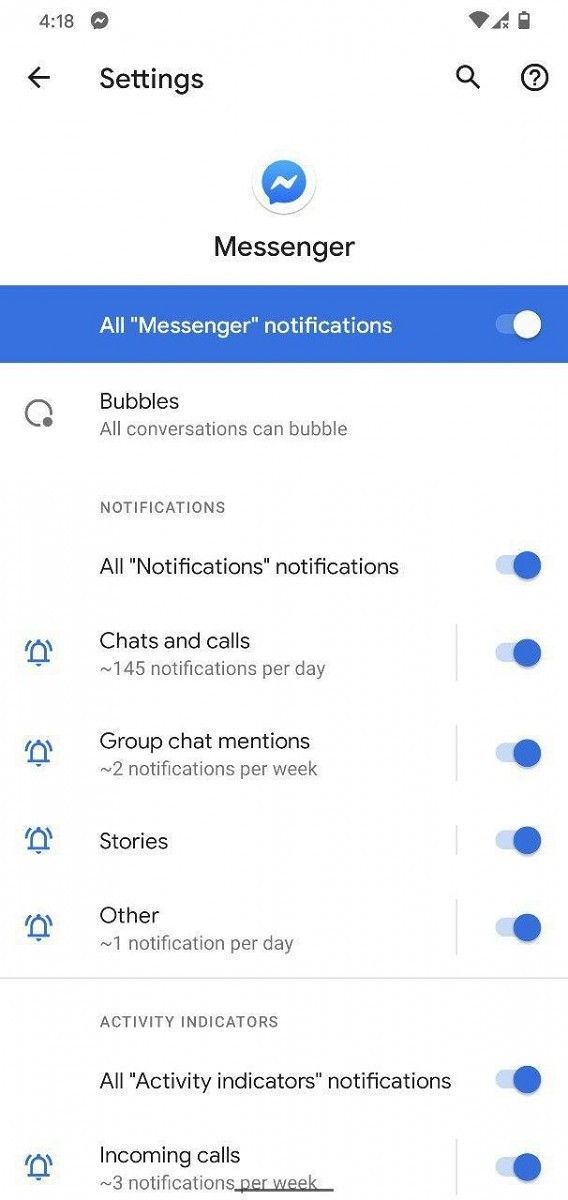Here is the cleaned-up and detailed caption:

"A screenshot of the settings interface for the Messenger app. The interface displays various notification preferences and options:

- The top bar shows a signal indicator with full Wi-Fi and full signal strength, but not a full battery. A left arrow, settings icon, magnifying glass, and question mark are also visible.
- Below this, there's a white circle with a blue Messenger icon and the text 'Messenger' in black.
- A blue bar reads 'All Messenger Notifications' with a toggle switch beside it.
- Under the notifications section, two categories are shown: 'Bubbles' and 'All Conversations Can Bubble', with toggles for enabling these features.
- Various notification preferences are outlined:
   - 'Chats and Calls': one notification per day (toggle switch)
   - 'Two Notifications a Week' (toggle switch)
   - 'Stories' (toggle switch)
   - 'Other': one notification per day (toggle switch)
- Text in gray indicates 'Activity Indicators', and in black, it states 'All Activity Indicators' with respective toggles for notifications.
- A section labeled 'Battle Icon and Call' mentions three notifications per week (toggle switch).
- The interface has a white background.

Additionally, another mention of the left arrow settings and magnifying glass is noted."